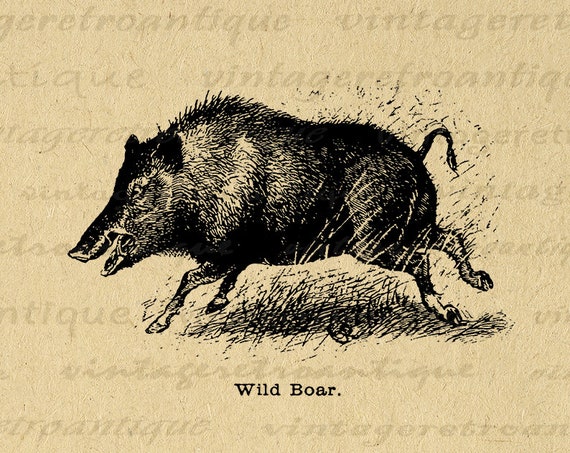A hand-drawn black ink sketch of a wild boar is set against weathered, light brown, tannish paper with a vintage feel. The boar is depicted mid-gallop, racing towards the left edge of the image. Its detailed features include a raised tail, forward-thrusting front legs, and backward-positioned back legs, indicating motion. The boar's open mouth reveals a visible tusk, and its humped back adds to its wild appearance. The background is adorned with various foreign words in a script font, such as geratronicu, vintagret, tecuv, and vintagrophantic, enhancing the old-world aesthetic. A shaded patch of grass beneath the boar shows blades flying into the air. Below the sketch, the label "wild boar." is printed in black text.